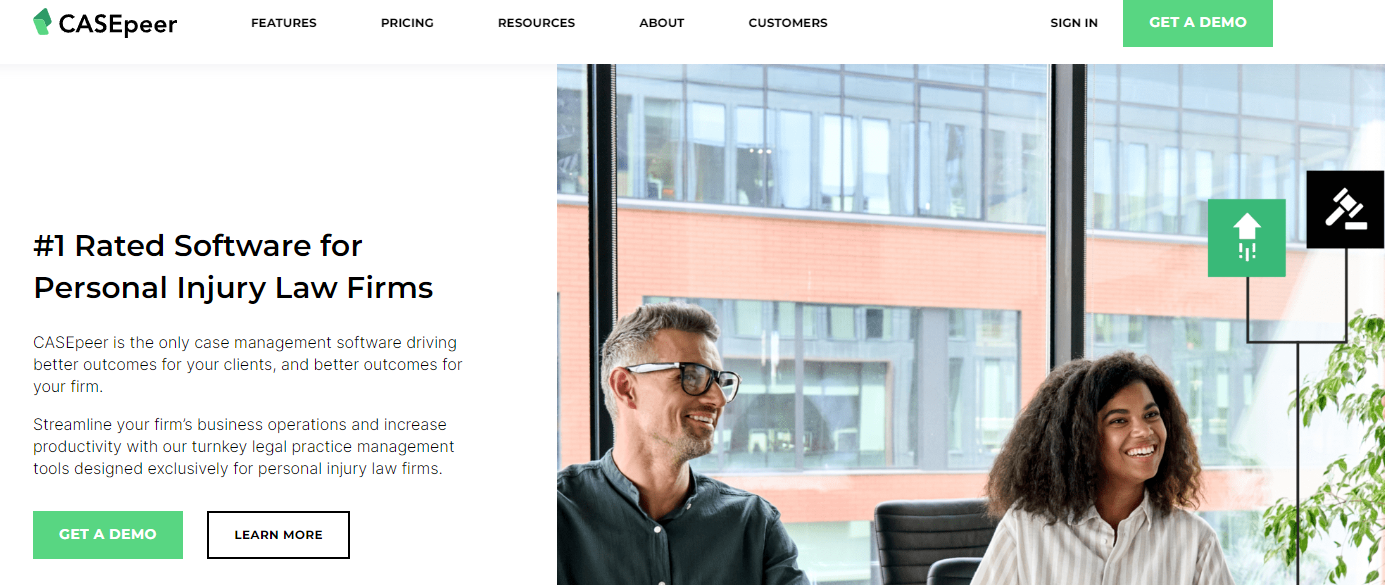The image displays a webpage with a clean white background showcasing a professional photo of a man and a woman seated in office chairs. The woman has large, curly textured hair and wears a button-down striped shirt, while the man sports short gray hair and a button-down gray shirt. Both individuals are looking to the right and smiling. Behind them, through large windows, a brick building with numerous windows is visible, enhancing the setting of a modern, well-lit office space. A leafy green plant is positioned to the right of the pair, adding a touch of nature to the scene.

The website is identified as "Casepeer," a legal practice management software platform. Prominent elements on the webpage include:
- A green box with an upward-pointing arrow.
- A black box featuring a gavel icon.
- A green folder icon on the left side of the image.

At the top, navigation buttons labeled "Features," "Pricing," "Resources," "About," and "Customers" are displayed, alongside a "Sign-In" button and a green "Get a Demo" button.

Text on the left side of the image proclaims: "Number one rated software for personal injury law firms. Casepeer is the only case management software driving better outcomes for your clients and better outcomes for your firm. Expand your firm's business operations and increase productivity with our turnkey legal practice management tools designed exclusively for personal injury law firms." Additional calls to action include a green "Get a Demo" box and a "Learn More" button.